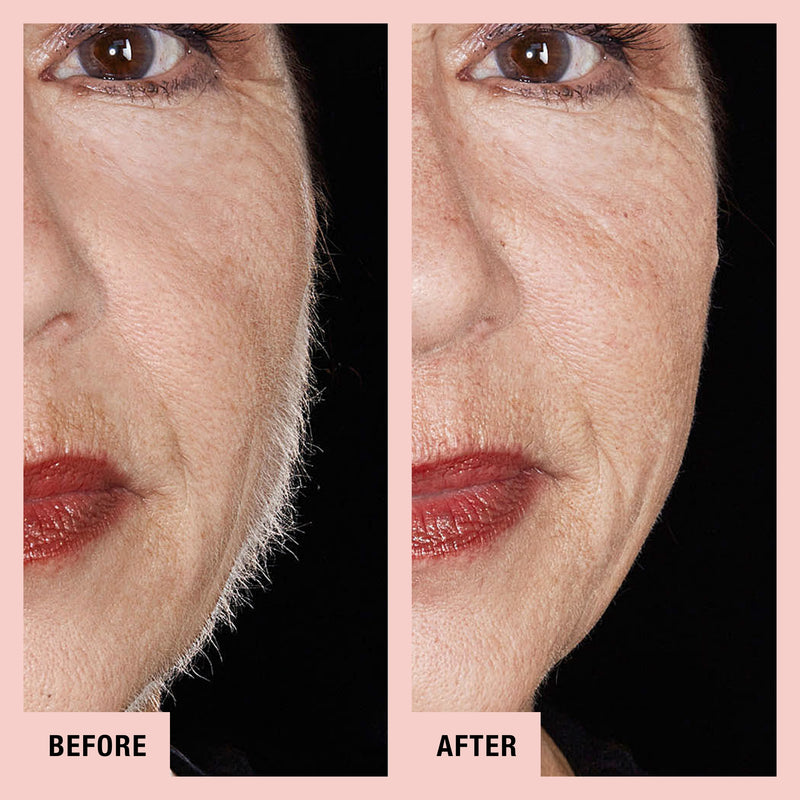The image is a vertically rectangular before-and-after photograph of a woman's face, divided into two equally sized sections, each framed by a thin pink border. The left side shows the "before" image, inside a pink box with black text reading "BEFORE" in the bottom left corner. This image reveals a close-up of the woman's left side of her face, featuring brown eyes, dark red (possibly reddish-orange) lipstick, and visible light gray hairs or white fuzz along her cheek and jawline. Her wrinkles are slightly visible and the photo is backlit, emphasizing the hair and giving a slightly shadowed effect.

The right side presents the "after" image, also featuring a close-up of the same side of the woman's face with a pink border. In this photograph, the light shines directly on her face, eliminating the visibility of the facial hair, making her skin appear smoother although her wrinkles are more pronounced. The woman retains the same dark red lips and brown eyes. The bottom left corner of this image reads "AFTER" in black letters. The set of photographs is set against a black background.